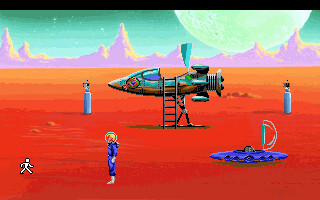The image captures a small, pixelated video game scene, evocative of a classic, retro gaming style. The setting is a desolate, orangey-red desert landscape that suggests a Martian environment. The background features a clear teal sky with a distinctive purplish-pink mountain range and the prominent lower half of a large, white moon positioned in the top right. Central to the scene is a silvery-blue spaceship with an open cockpit, which resembles a small rocket ship. A ladder extends from the ground to the spacecraft's hatch. To its right is a smaller, blue UFO-style alien craft with a semi-circular glass cockpit also open. In the foreground stands an astronaut, donned in a blue suit with a clear round helmet and yellow hair, gazing towards the left. Silver fuel tanks flank the rocket ship. Additionally, a tiny stick-figure-like image appears to be walking towards the astronaut, adding a curious detail to this captivating, interstellar scene.